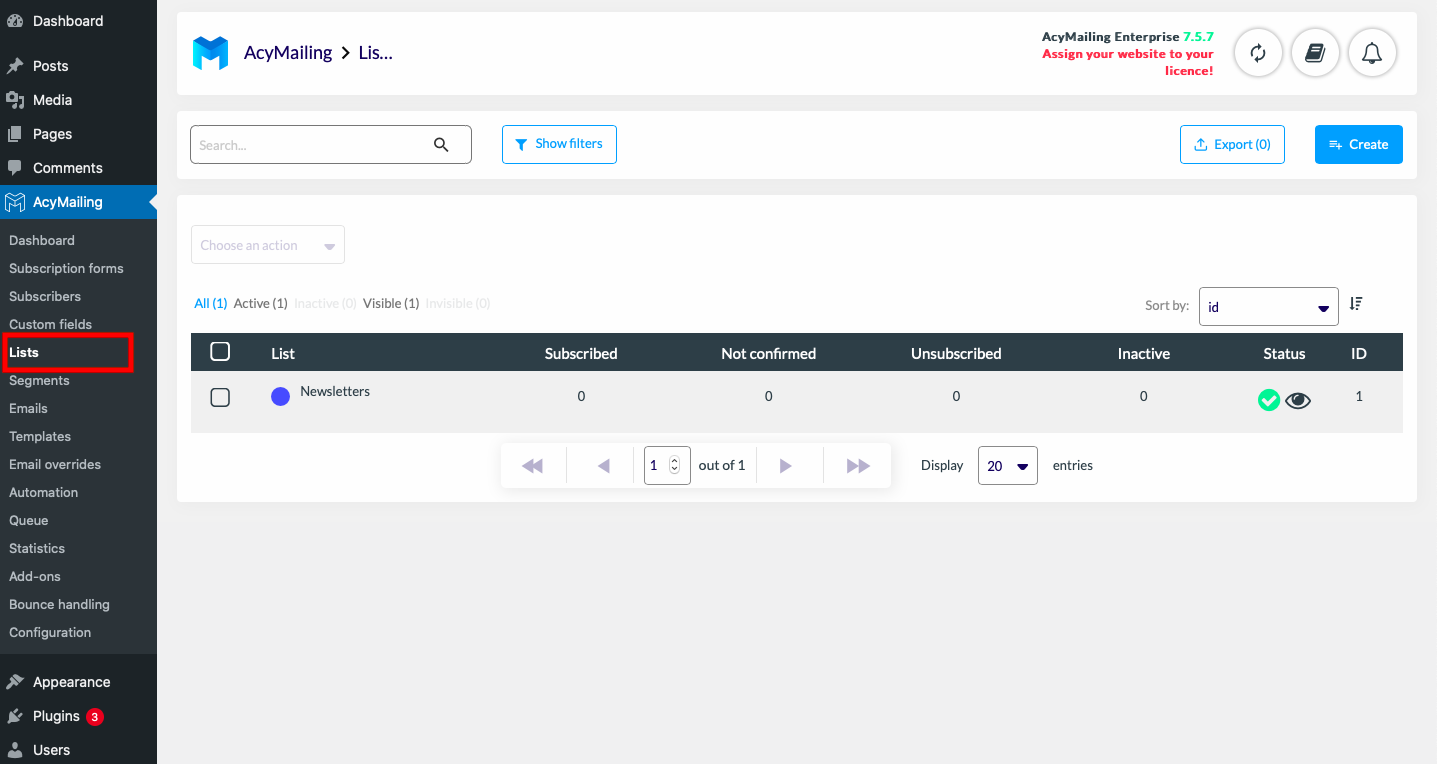The image showcases the user interface of the AC Mailing Enterprise's website. Prominently located in the top-left corner is the company’s logo, indicating the brand identity. In the top-right corner, the text "AC Mailing Enterprise" is displayed along with a version number, which appears to be 7.5.7, written in a green font that is somewhat difficult to discern.

The interface includes several interactive icons located at the top: a book link, a notifications button, and a refresh icon. Central to the screen is a search facility equipped with filtering and export options, allowing users to create custom searches.

The search results are presented in a tabular format, with column headers such as "List," "Subscribed," "Not Confirmed," "Unsubscribed," "Inactive," "Status," and "ID." These columns facilitate easy filtering and categorization of the data.

On the left-hand side of the screen, a grey panel functions as a dashboard with various navigational headings. The currently selected section is "AC Mailing," highlighted in blue. Further down is the "Lists" section, emphasized by a red rectangle likely indicating it is the active view at the moment, specifically focusing on AC Mailing lists. This section allows users to create and manage their mailing lists.

Toward the bottom of the panel, the "Plugins" section is marked, noting the presence of three configured plugins by displaying the number three next to it.